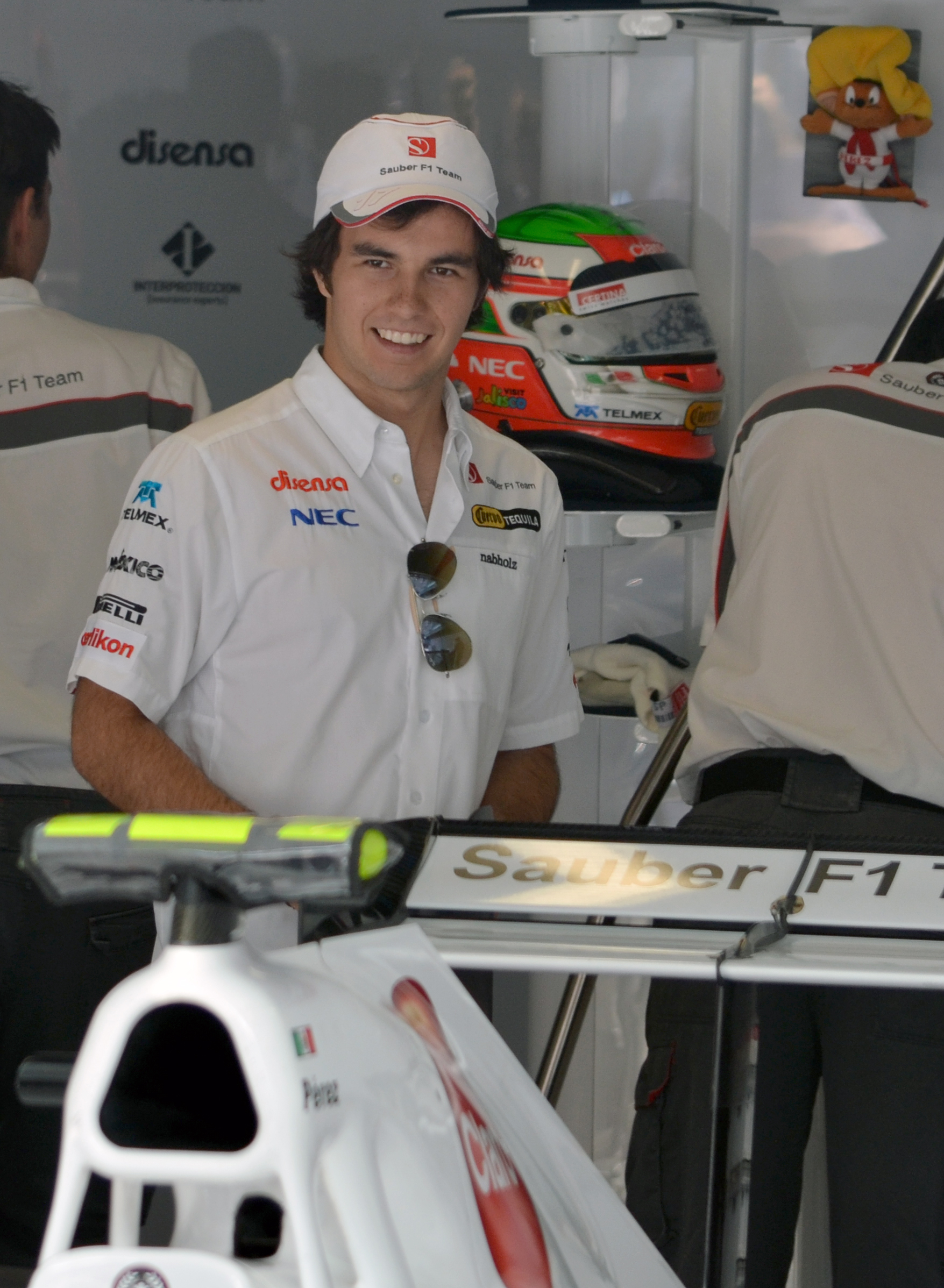In the image, a young man, potentially an F1 racer, stands smiling, drawing the viewer's attention. He is wearing a white cap emblazoned with "Sauber F1 Team" and a white, short-sleeved polo shirt adorned with numerous sponsor logos, including NEC, Mexico, Elicon, Nables, and possibly something related to tequila. His short brown hair peeks out from under the cap. Sunglasses are tucked into the button-up area of his shirt. Surrounding him are several other men in similar white polo shirts and gray pants, with their backs turned or partially visible. A red, green, and white helmet can be seen in the background, adding to the motorsport ambiance. The setting appears to have a white background, with some kind of bar or structure in the foreground.